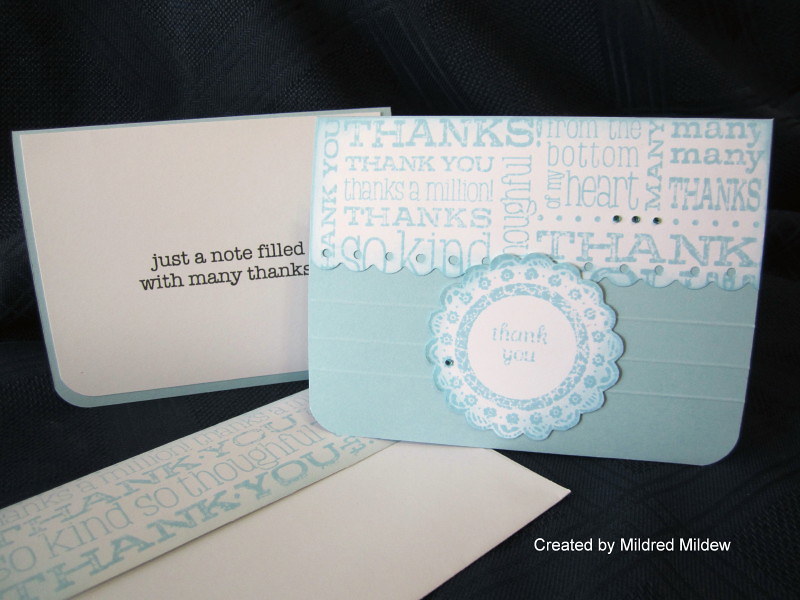This photograph features three intricately designed stationary items arranged against a navy backdrop. Dominating the scene, a rectangular, light blue note or envelope with frilly white edges and a decorative circular badge at the center that reads "Thank you." The upper half of this item features an array of "thanks" and "thank you" messages in various fonts and directions, creating a dynamic pattern. Adjacent to this, on the left, is a white card with rounded corners that states, "Just a note filled with many thanks" in elegant black font. The card's matching white envelope, detailed with light blue text repeating similar gratitude phrases, lies at an angle with its flap open, hinting at the cohesive design theme of the set. In the bottom right corner of the image, the text "Created by Mildred Mildew" is prominently displayed, attributing the creator.